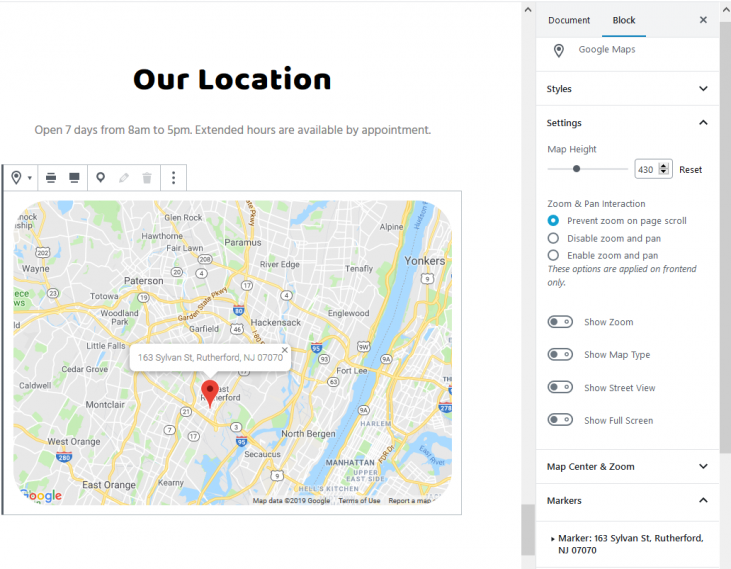**Caption:**

The image captures a detailed screen of a Google Maps interface displaying the New York City area, with specific focus on Yonkers, Manhattan, and surrounding regions. A red location pin marks the address 163 Sylvan Street, Rutherford, New Jersey, 07070. The map view is dated with a copyright year of 2019, and users can see terms of use and reporting options.

On the left side of the image, against a white background, there is text stating "Our Location" and operational hours: "Open seven days from 8 a.m. to 5 p.m. Extended hours are available by appointment." Adjacent icons such as a printer, computer, and additional location pins are visible.

The right side of the image features a dropdown menu under the sections "Document" and "Block," with a blue line highlighting the "Block" section. It shows a black "X," a gray location pin labeled "Google Maps," and submenus including "Style" with a dropdown menu, "Settings" with another dropdown menu, and "Map Height" with a setting at 430 and a 'reset' button. Further down, the "Zoom and Pan Interaction" section has the option "Prevent Zoom on Page Scroll" checked in blue, with unchecked options for disabling and enabling zoom and pan.

Additional checkboxes for "Show Zoom," "Show Map Type," "Show Street View," and "Show Full Screen" are visible in gray. Lastly, the section "Map, Center, and Zoom" and "Markers" lists a marker for 163 Sylvan Street, Rutherford, New Jersey, 07070.